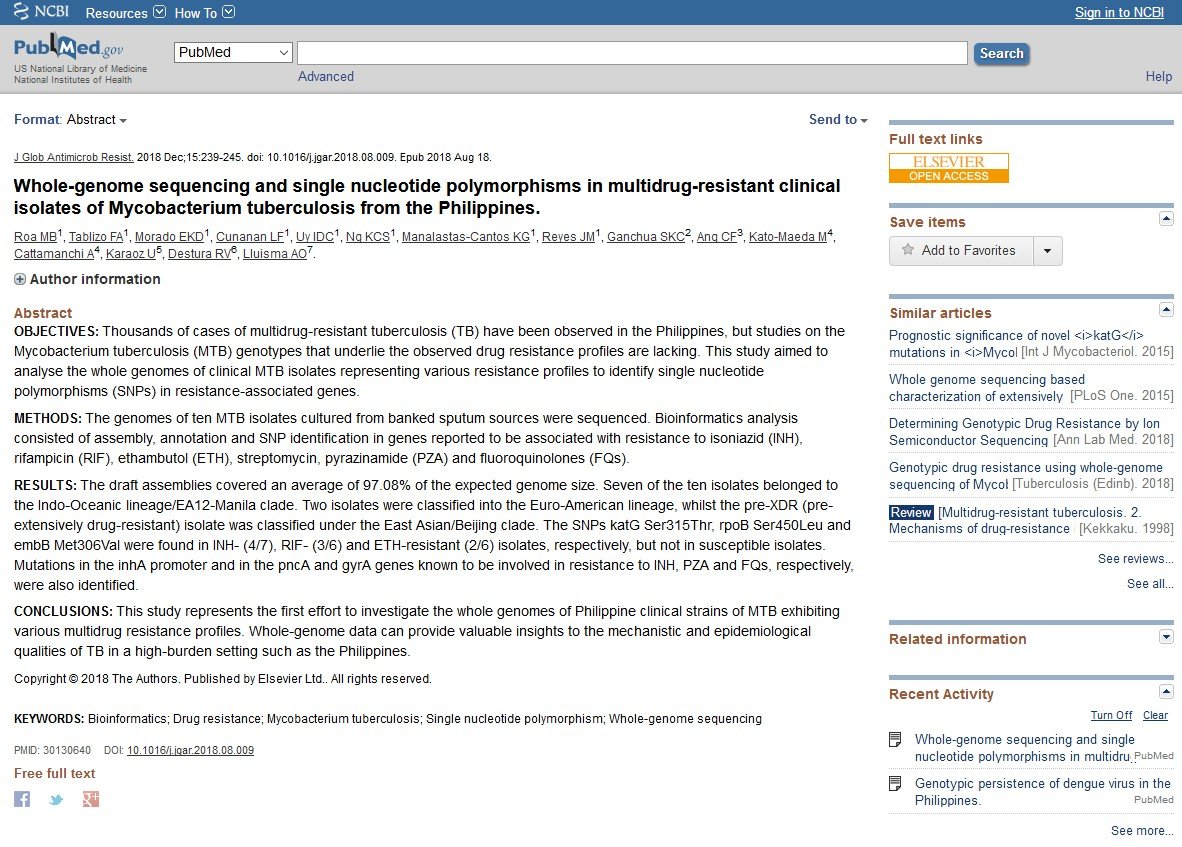A screenshot from the PubMed.gov website showcases an academic article listed under the U.S. National Library of Medicine, National Institutes of Health. The article, dated December 15, 2018, and first published on August 18, 2018, is prominently titled in bold black text: "Whole-genome sequencing and single nucleotide polymorphisms in multidrug-resistant clinical isolates of Mycobacterium tuberculosis from the Philippines."

The abstract of the article is segmented into clear sections—objectives, methods, results, and conclusions. On the right side of the screen, several options are visible for accessing additional resources: full-text links via Elsevier, open access, save items, and similar articles. Five similar articles are listed, followed by sections for related information and recent activity, both located in the lower right-hand corner.